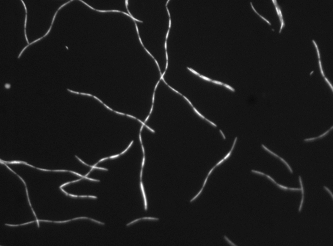The image depicts an abstract design on a solid black background, featuring numerous white, squiggly lines with frequent breaks in them. These lines vary in direction, crossing over each other and sometimes branching off, creating a complex web-like pattern that covers the entire image. The white lines, although irregular and seemingly random, give the impression of a magnified view of an organism or a computer-generated design. There is no text or other objects present in the image, and the only colors seen are black and white. The setting or origin of the image is ambiguous, but it evokes the appearance of either a microscopic view of a worm or parasite or an artistic rendition made with digital tools.